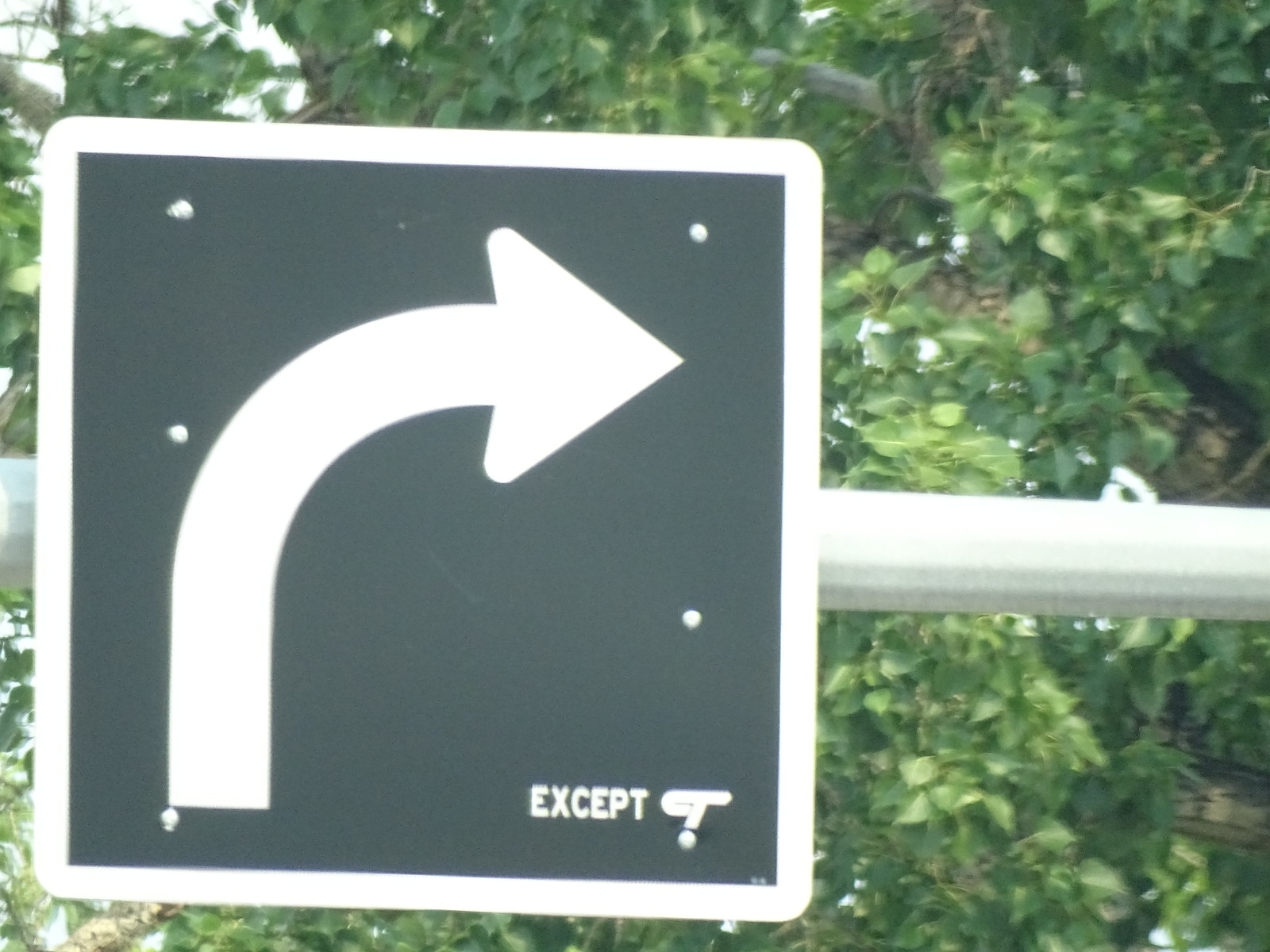A man is signaling to turn right at an intersection, specifically indicating that the turn should be made, except in the case of a traffic stop. The sign accompanying him is black and white and reiterates the instruction, advising drivers to turn right unless directed otherwise by a traffic stop.